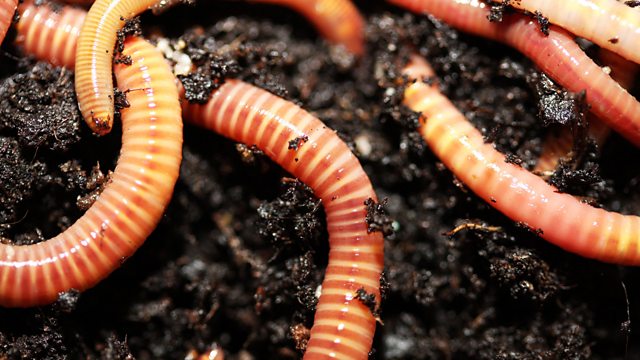This close-up image captures a group of healthy earthworms entwined in moist, dark brown to almost black soil. The earthworms are vividly detailed, revealing their pinkish or reddish-orange bodies adorned with distinct, well-defined rings that appear white or yellowish. There seems to be at least six worms in the image, their bodies partially covered by the damp soil they are immersed in. The worms display varied stripe patterns along their lengths, with some showing more pronounced stripes and others with slightly faded ones. The intricate details allow for a clear view of the worms' textures, indicating their robust and moist appearances as they navigate through the rich earth.